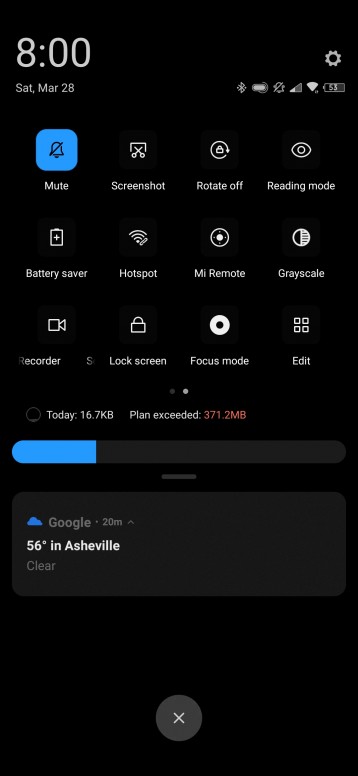**Caption:**

This screenshot, captured in dark mode, features a solid black background with white text and various icons. At the top left, the time is displayed as 8:00, followed by a small gray label indicating it is Saturday, March 28. Adjacent to the time is a settings icon resembling a gear. Various phone status symbols are aligned to the right, including a Bluetooth emblem, a battery icon indicating 53% charge, a bell icon with a cross through it signifying mute, cellular signal bars, and a Wi-Fi symbol.

The image also includes a series of settings and icons extending halfway down the screen. The first icon is light blue, labeled "Mute," and features a bell with a cross. Following that is the "Screenshot" icon, pictured with scissors, though it is not highlighted. Other icons include "Rotate Off" (a circle with a lock), "Focus Mode" (an eyeball symbol), "Battery Saver" (a battery with a plus sign), "Hotspot" (a Wi-Fi signal), "MI Remote" (a circle with a dot inside), "Grayscale" (a circle divided into black and white halves), "Recorder" (camera icon), "Lock Screen" (lock icon), "Focus Mode" again (white circle with a black dot), and "Edit" (four small squares).

Below this section, there is brief information indicating recent activity: "Today, 16.7 KB," and a notice of exceeded data usage: "Plan exceeded 371.2 MB." A blue progress bar, filled about one-third of the way, is positioned underneath these details.

Further down, a gray box displays more specific information: "Google, 20 minutes," paired with a blue cloud icon. Additionally, the current weather is noted as 56 degrees in Asheville with clear conditions. The bottom part of the screenshot shows two dots, one highlighted and one grayed out, suggesting navigation indicators for additional settings or panels.